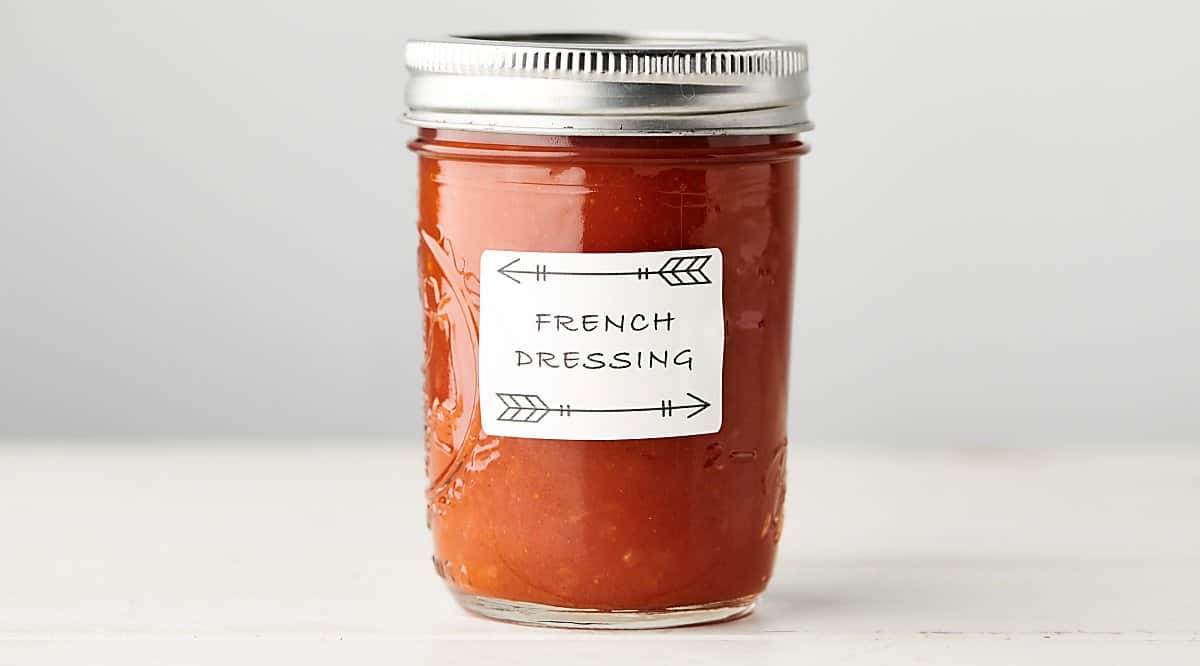The image displays a small, cylindrical mason-style jar, likely a jelly jar, with a capacity of six to eight ounces, resting on a white surface against a blurred pale gray background. The jar is made of thick glass with multiple layers at the bottom and features a circular imprint of vines and flowers on the left side and measurements on the right. Adorning the jar is a piece of white paper labeled "French Dressing" in black print, accompanied by two feathered black arrows—one at the top pointing left and one at the bottom pointing right. The jar is sealed with a silver metal screw-top lid, and it contains an orange-red liquid, presumably French dressing.